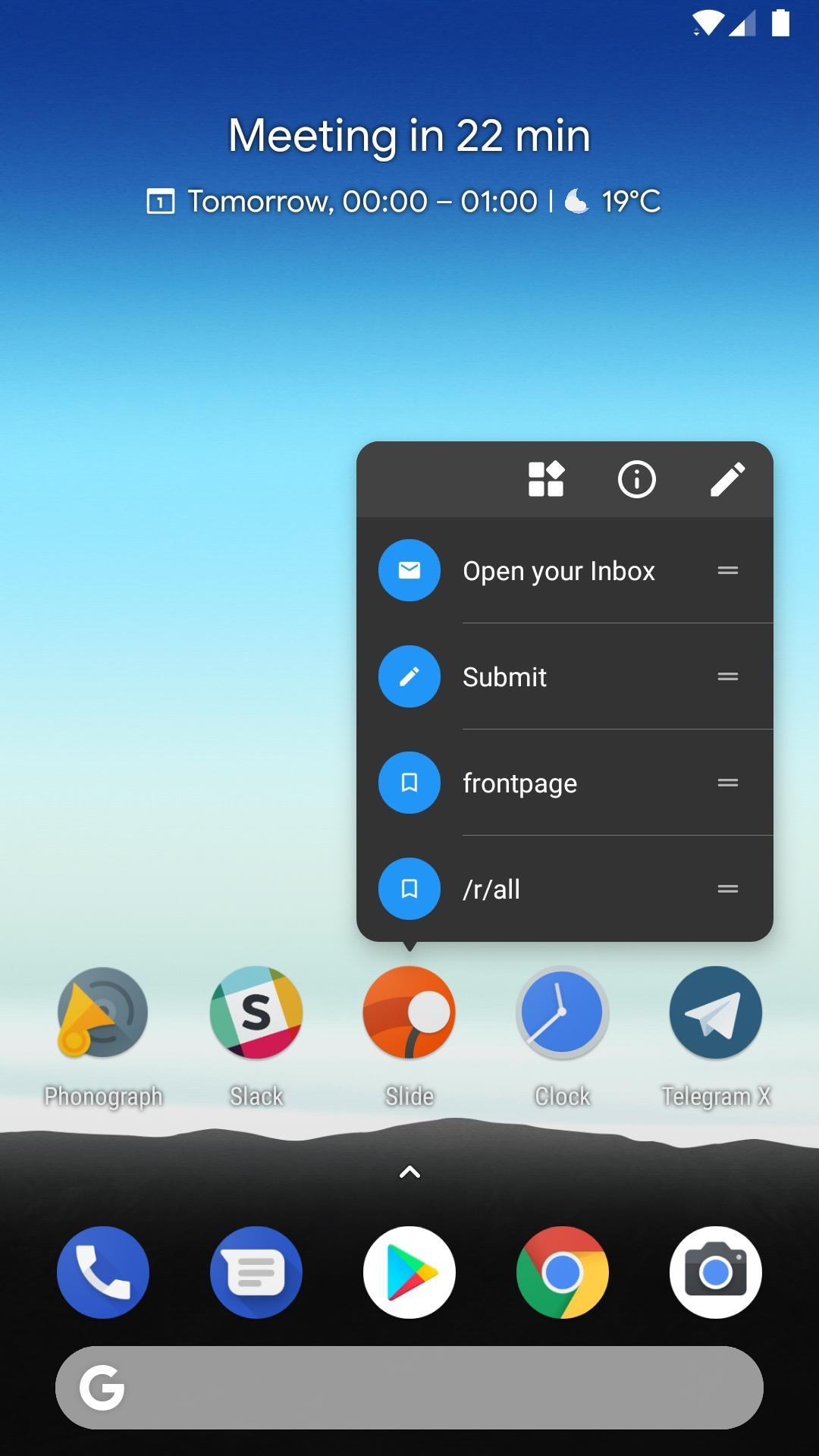The image depicts the home screen of a digital device, likely a smartphone or small tablet. The interface is populated with a variety of colorful app icons, primarily clustered towards the bottom of the screen. The prominent app icons include a phonograph icon, Slack, Slide, Clock, and Telegram. Below these, additional icons for various essential apps such as the Camera, Phone, and Chrome Browser are visible. 

At the very bottom of the screen is a search panel allowing users to enter a Google search query. The upper portion of the screen features a notification banner in white text against a blue background, indicating an upcoming meeting in 22 minutes and the current temperature being 19 degrees Celsius.

Centrally positioned but slightly to the right is a small, grey floating dialogue window offering further options like "Open Your Inbox," "Submit," "Front Page," and several others which appear to function as an editor or bookmark manager.